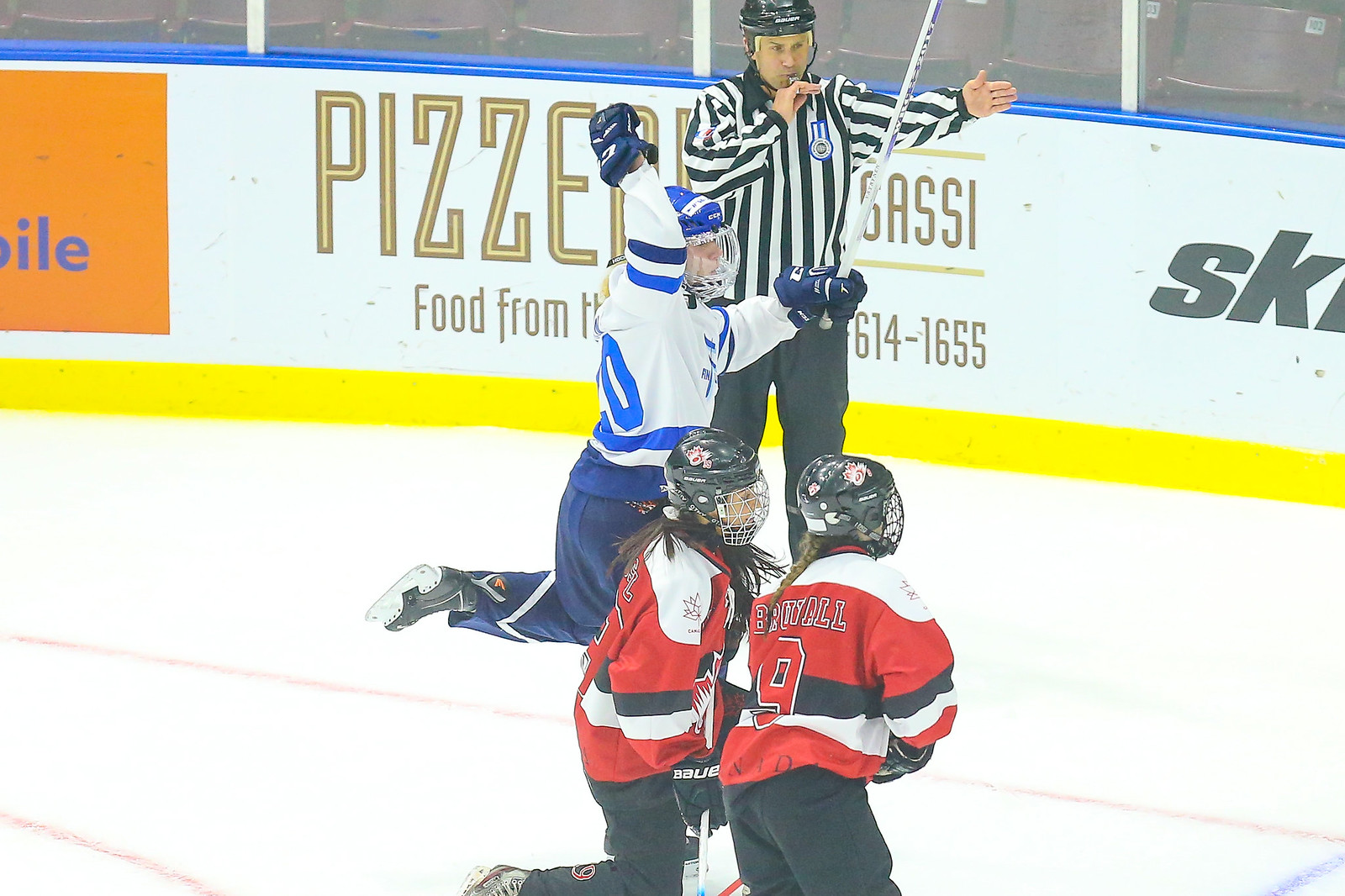The image captures a dynamic moment on a hockey rink showing three hockey players and a referee on the white ice. The two players closest to the camera are wearing black pants and red, white, and black jerseys with black helmets accented in red and white. One of these players has long dark hair reaching their shoulders, while the other sports a long braid going down to mid-back. These players also seem to have text and numbers on their jerseys, with visible details suggesting the name "Brunal" and the number nine. A bit further back, an opponent is clad in blue pants and a predominantly white jersey adorned with light blue and dark blue stripes, complemented by a blue helmet. The referee, situated in the background, is donned in dark pants and a classic black-and-white striped shirt, caught in the act of blowing his whistle with one hand extended. The rink's wall, painted white with a blue stripe on top and a yellow stripe at the bottom, features some advertisements, including partially readable golden lettering that spells out "pizzeria."